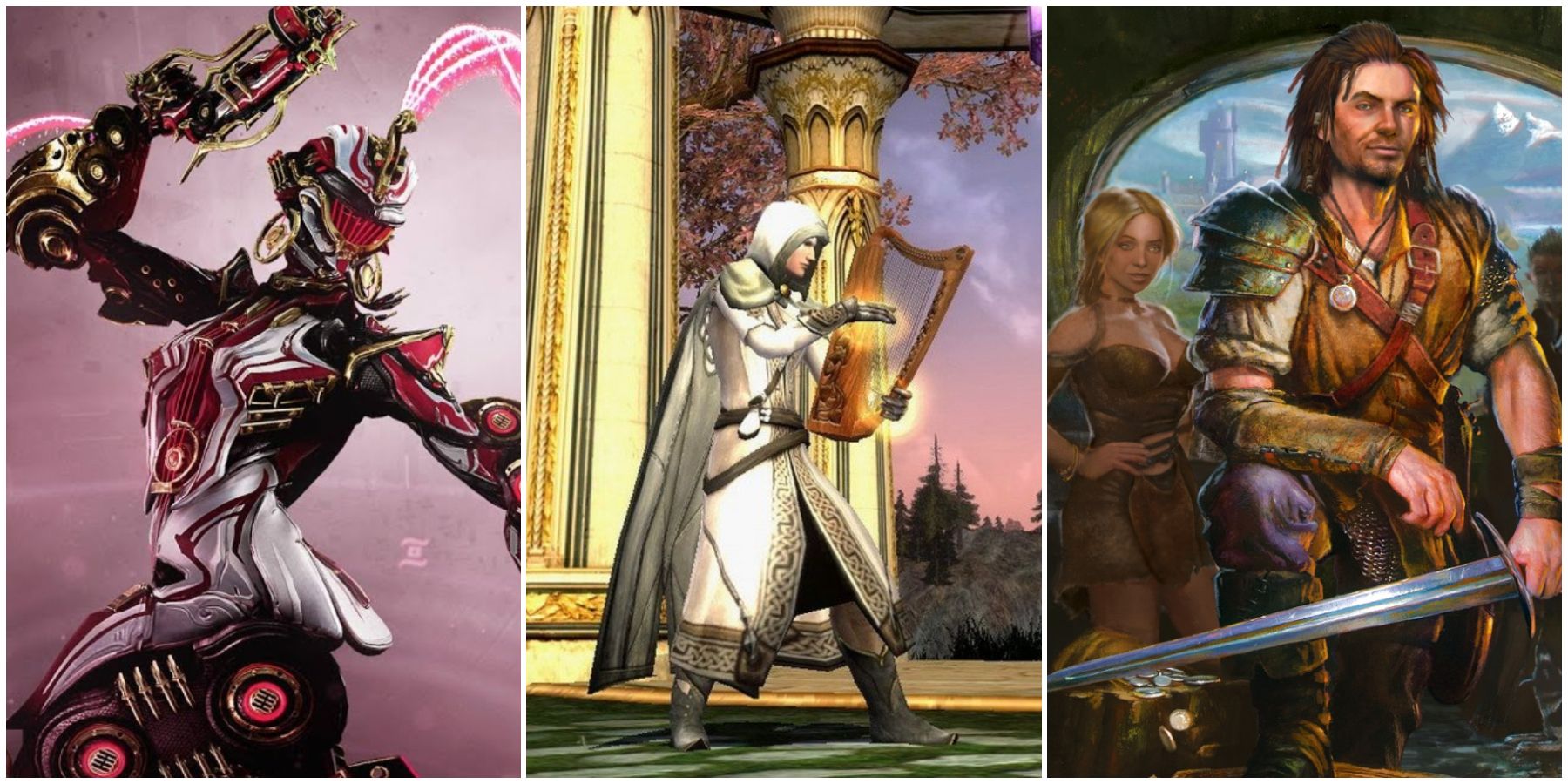The image consists of three side-by-side panes, each showcasing computer-generated scenes from video games. 

- The rightmost pane features a roguish knight-like character kneeling and facing the viewer, holding a sword. Behind him stands a young woman in a low-cut top, also looking towards the viewer. The backdrop reveals an open landscape window, displaying majestic mountains.

- The center pane depicts a cloaked figure clad in gray and white attire, with only his face visible. He cradles a golden harp in his hands. The setting is an opulent gold room, highlighted by a golden pillar and a distant landscape seen through the background.

- The leftmost pane presents a mechanical, female robot, with her body twisted and one arm raised. She is glancing over her shoulder.

Each pane offers a unique and captivating visual narrative, blending detailed character design with immersive environments.